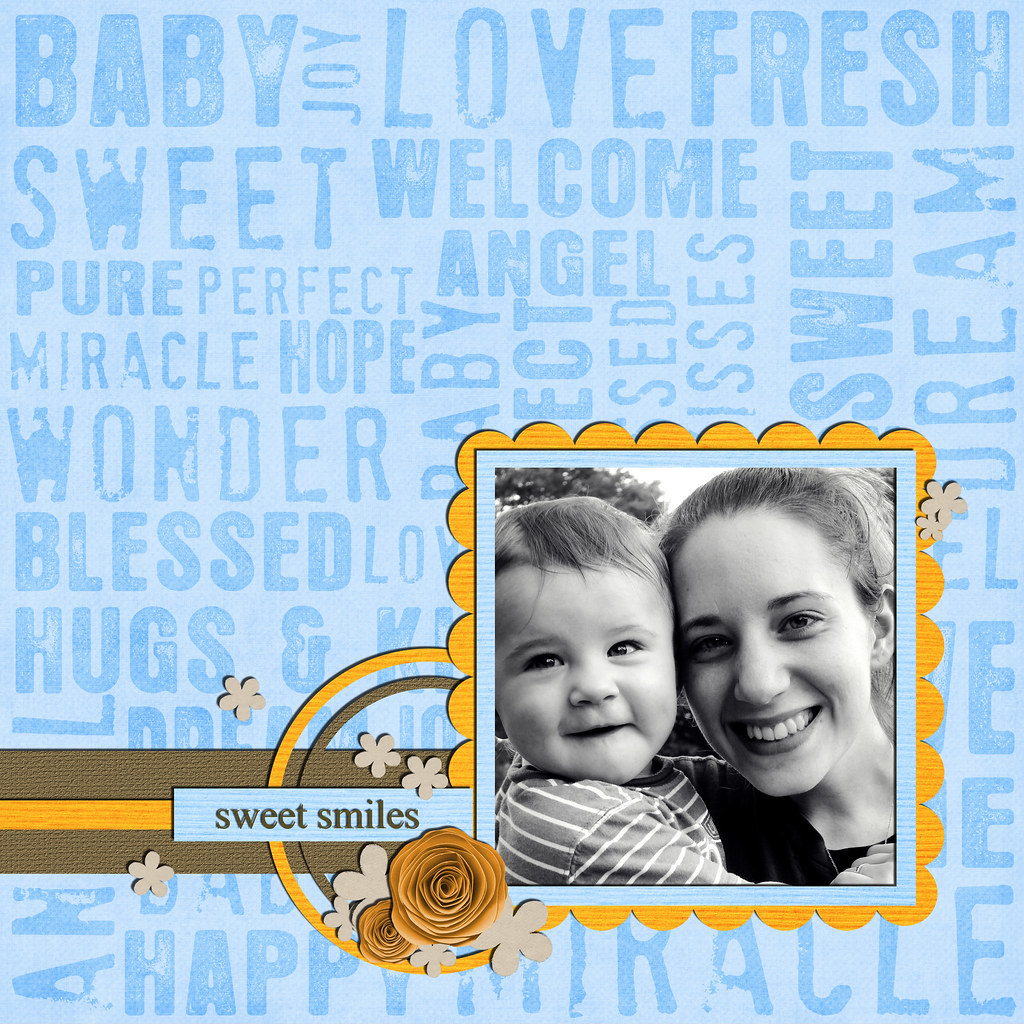The image appears to be a personalized baby card with a retro aesthetic, resembling the cover of an old record album or an album cover from a DVD or CD. The background is a light blue canvas adorned with an array of words such as "baby," "joy," "love," "fresh," "sweet," "welcome," "angel," "wonder," "blessed," "hugs and kisses," "happy," "miracle," and "dream," creating a vibrant collage in darker blue, running both vertically and horizontally.

Prominently positioned on the bottom right is a black-and-white photograph of a young woman and a toddler. The close-up shows them from the shoulders up, both smiling directly into the camera. The woman, likely in her early to mid-20s, is gently leaning her head against the boy, who wears a dark long-sleeved shirt with white horizontal stripes. Both subjects have light skin and light-colored hair. Surrounding the photo is a decorative yellow scalloped border with floral and clover elements. The phrase "sweet smiles" is seen in block lettering at the bottom left of the photo, adding a tender touch to the overall composition.